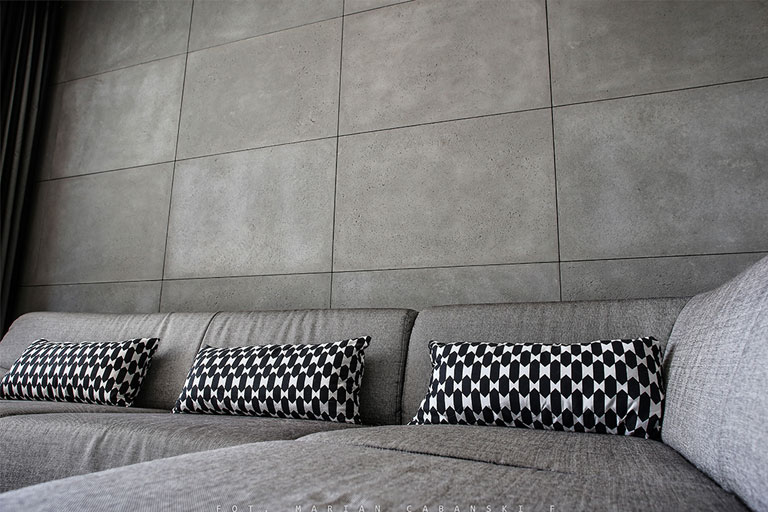The photograph captures a contemporary interior featuring a light gray L-shaped sectional couch made of either tweed or polyester fabric. The perspective is from on the couch, emphasizing its expansive design. Resting against the back of the couch are three identical black and white rectangular pillows with a bowtie checkered design. The backdrop of the scene is a light gray concrete wall segmented into large squares, contributing to the modern aesthetic. On the left side, a dark gray curtain or column is partially visible. The bottom of the image bears white text that reads "F-O-T M-A-R-I-A N C-A-B-A-N-S-K-I-F." The overall color palette is dominated by shades of gray, accentuated by the monochromatic pillows, adding to the sleek, cohesive vibe of the space.